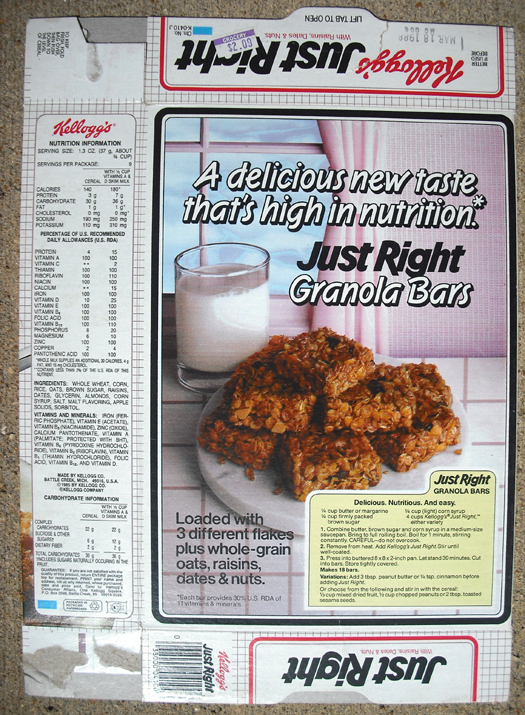This is a detailed photograph of a vintage Kellogg's Just Right granola bar box, displayed in a portrait orientation. The box features a prominent message stating, "A delicious new taste that's high in nutrition. Just Right Granola Bars." The front of the box showcases a photo of six granola bars arranged in a circular pyramid formation on a plate, accompanied by a glass of milk. The scene is set against a backdrop of a pink and white tiled countertop, with a sunny window framed by pink curtains. The white box background includes a price sticker labeled $2.09. It appears that the box has been opened and laid flat, revealing the nutrition facts to the left, listing calories, fats, vitamins, and ingredients. Additionally, there is a recipe for the granola bars on a yellow index-style card located below the image. The iconic red Kellogg’s logo is positioned at the top, along with large, bold black letters spelling "Just Right." The box also features an expiration date at the top and a UPC barcode at the bottom. The background of the overall setting includes a grey and brown rug.